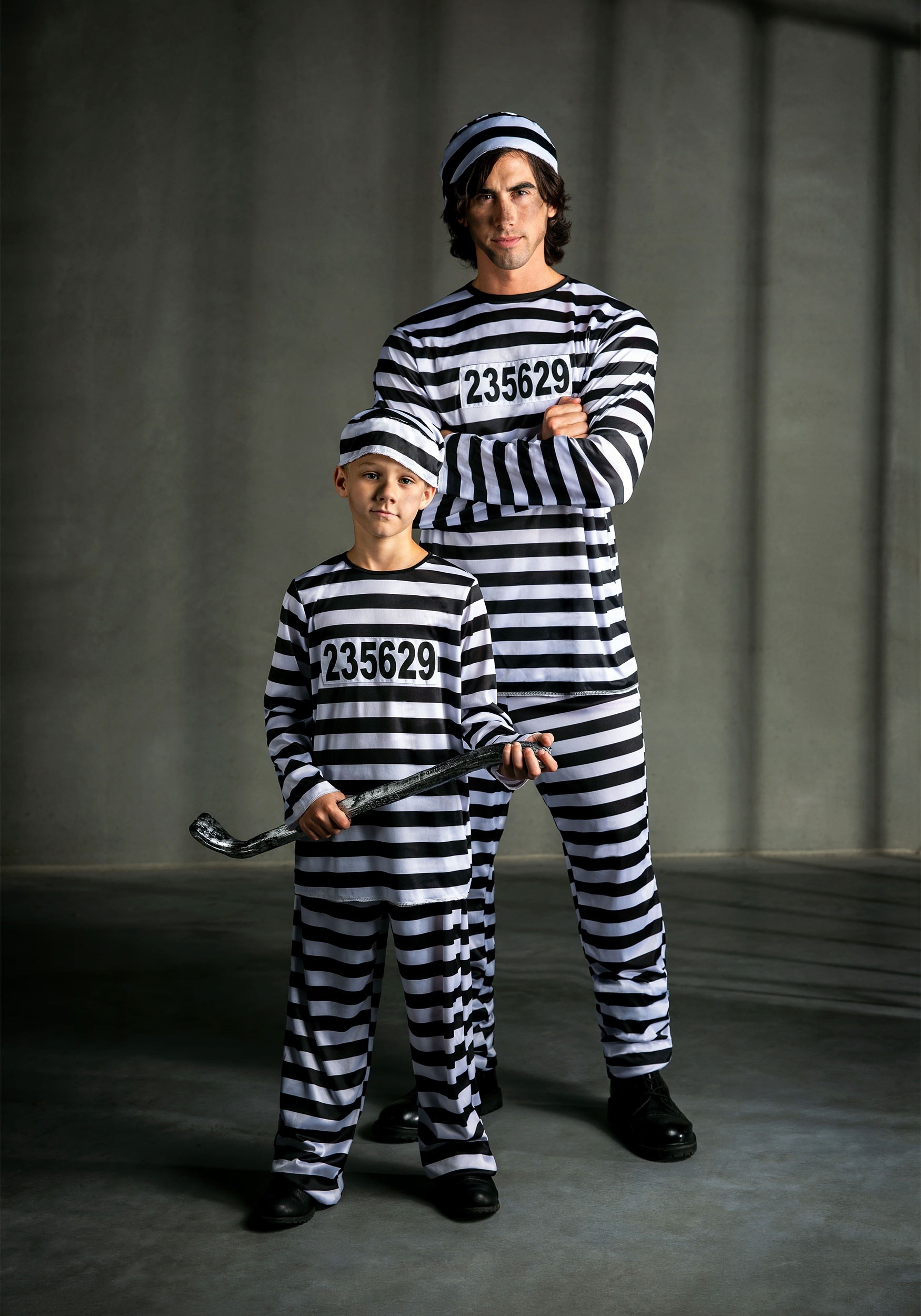This image features a young man and a middle school-aged boy, both dressed in distinctive prison-style uniforms characterized by horizontal black and white stripes. The young man, likely in his twenties, has dark brown, shaggy hair and a stern facial expression. Standing behind the boy with his arms crossed, he gives off a protective yet intense air. The boy, appearing approximately eight years old, holds a black crowbar in his hands and shares the same serious demeanor as the man behind him. Both are adorned with matching numbers "235629" on white bibs on their chests, further accentuating their prisoner personas.

They both wear identical black and white striped caps and black shoes, completing their coordinated outfits. The setting of the image evokes a prison environment, with a dark gray floor and a gray backdrop. Light coming in from the right side casts strong shadows that resemble prison bars on the wall, reinforcing the overall motif. The atmosphere, costumes, and expressions create a highly detailed and evocative depiction of the prisoner theme.